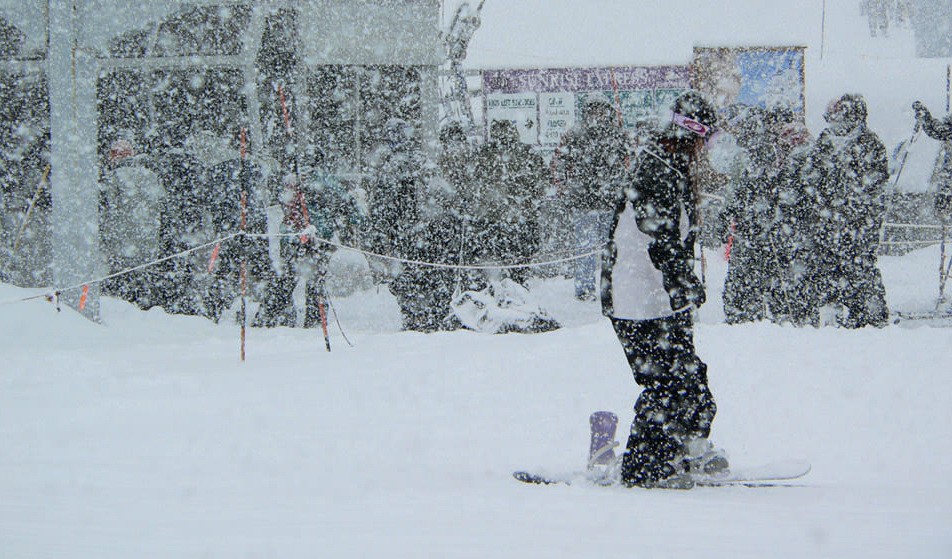The image captures a bustling scene during a heavy snowstorm, most likely outside at a ski area or snow event. At the forefront, slightly to the right of center, stands a person on cross-country skis or possibly a snowboard. They're clad in a black and white coat, black snow pants, and a snow cap, with pink goggles adding a splash of color. The heavy snowfall creates large, blurring flakes that obscure finer details. Behind this individual, a rope comes up and crosses from the middle left behind them, sectioning off a small area.

The background is populated with numerous people dressed in full snow gear, presumably waiting in a line to enter a building for shelter, food, or supplies. The building to the left has visible glass windows and possibly a banner or billboard with indistinct white writing. The sky is a murky gray, adding to the blizzard's intensity, making the entire scene look gray and snowy with flurries filling the air. The overall mood is one of cold, intense weather with people actively braving the storm.